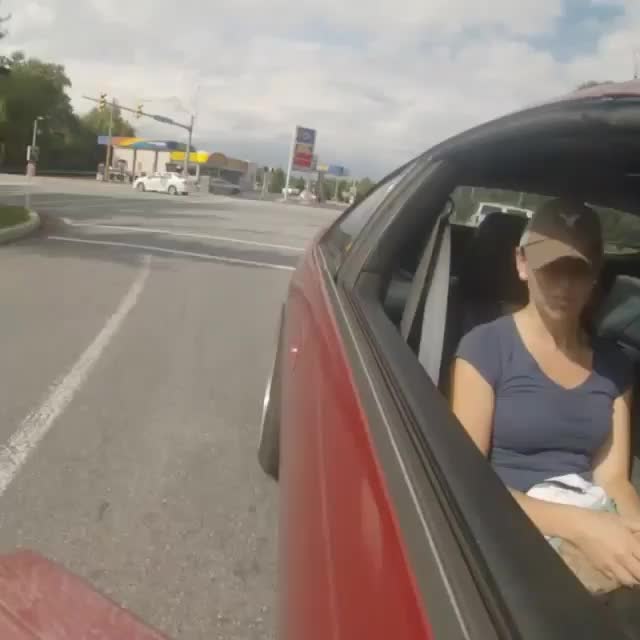The photograph captures a detailed scene of a red car traveling along a highway on a cloudy afternoon. The car, which has black lines outlining its windows and a prominent black wheel at the rear, is moving towards the bottom right corner of the image. Inside the car, a fair-skinned woman is visible. She is wearing a brown baseball cap with a white bird logo on the front and a blue t-shirt. She appears to be looking downward while holding a grey object, and she is secured with a grey seatbelt. The car is surrounded by a road with white markings, indicating lane divisions, and there are several street road signs in red, yellow, and blue colors visible at the center top of the picture. Overhead traffic lights are mounted on a horizontal pole, adding to the urban setting. In the distance, there are some cars partly obscured by rubble, and structures resembling a garage with overhead areas and possibly pumps. The sky is mostly cloudy, but patches of blue can be seen, suggesting variable weather conditions.